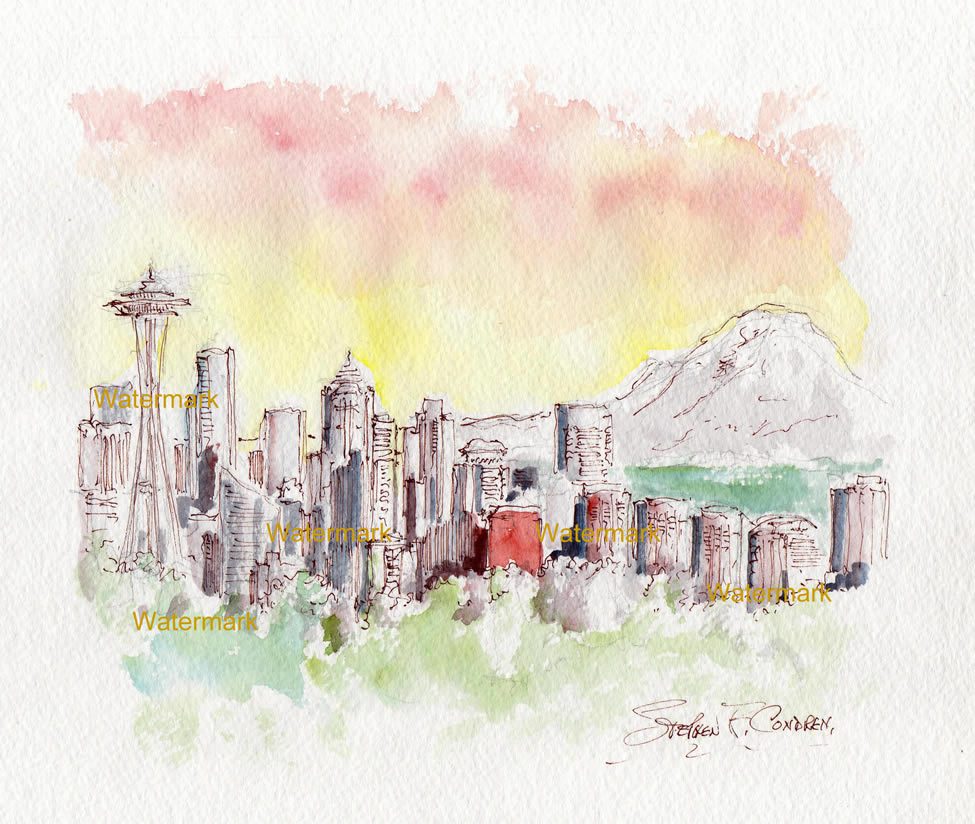This detailed watercolor illustration, signed by F. Condren, depicts an impressionistic cityscape against a dreamy pastel sky. The background of the artwork transitions from a light gray at the very top, blending into shades of pink and pale white clouds, culminating in a vivid red and yellow horizon that suggests either sunrise or sunset. A prominent hill or mountain, painted white, rises in the backdrop on the right side of the paper.

In the lower right corner, hints of greenish water or grass are visible, adding a touch of nature to the urban environment. The city's skyline features approximately twenty skyscrapers of varying sizes, rendered in a wobbly and abstract style with a notable lack of detail, enhancing the dreamy quality of the scene. Among the buildings, a tall structure resembling the Space Needle stands out prominently on the left side.

The foreground contains more green foliage, suggesting a park or natural area within the city. Superimposed over the entire image are yellow words reading "watermark," repeated throughout, indicating the nature of the digital watermark. The illustration covers about 75% of the white paper, leaving some negative space to emphasize the coloration and form of the elements within.